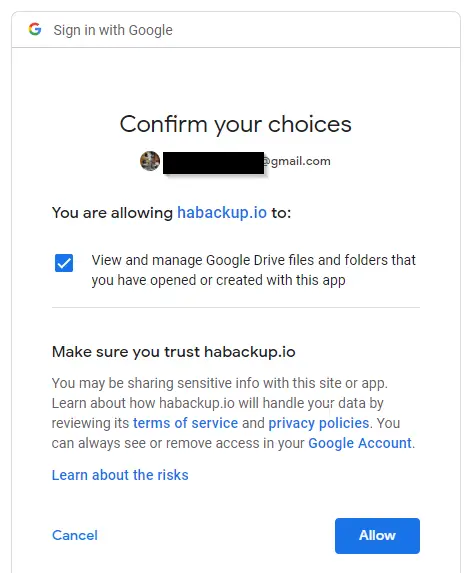A screenshot of a Google sign-in page is presented. At the top of the page, there is the text "Sign in with Google." Below is a section to enter the Google ID. Above this input field, the phrase "Confirm Your Choices" is prominently displayed. Further down, a message reads: "You are allowing user habacup.io to view and manage Google Drive files and folders that you have opened and created with this app." A cautionary note follows, stating: "Make sure you trust this user." Additionally, a clickable option labeled "Learn about the risks" is provided for more information. At the very bottom of the page, there are options to either cancel the action or, on the far right, a blue "Allow" button to proceed.